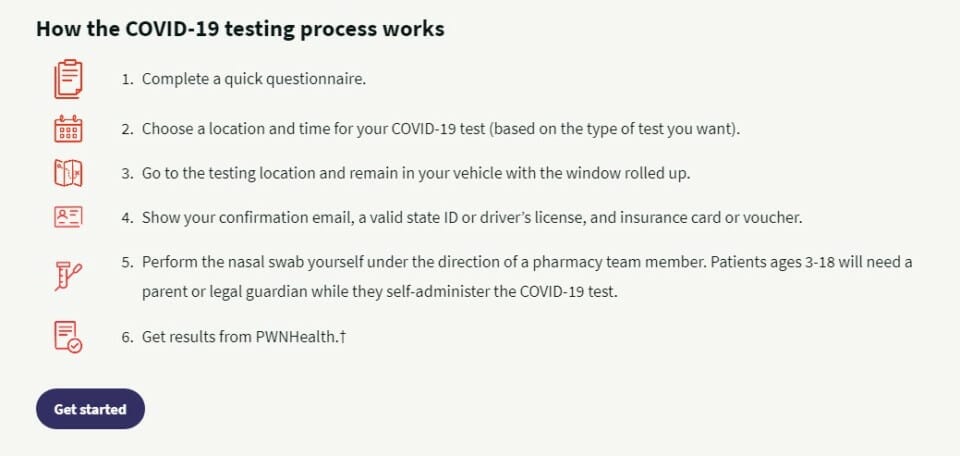The image features a light gray rectangular box with a black, bold heading stating, "How the COVID-19 Testing Process Works." Below the header, the process is outlined with numbered steps accompanied by icons:

1. A red clipboard icon with the text "Complete a quick questionnaire."
2. A calendar icon indicating, "Choose a location and time for your COVID-19 test," followed by the note, "based on the type of test you want."
3. A map icon labeled, "Go to the testing location; remain in your vehicle with the window rolled up."
4. An ID card icon with instructions to, "Show your confirmation email, a valid state ID or driver's license, and insurance card or voucher."
5. Instructions to "Perform the nasal swab yourself under the direction of a pharmacy team member," noting that "adults ages 3 to 18 will need a parent or legal guardian while they self-administer the COVID-19 test."
6. A concluding statement, "Get results from PWN Health."

Each step is clearly numbered and visually supported by relevant icons for easy understanding.